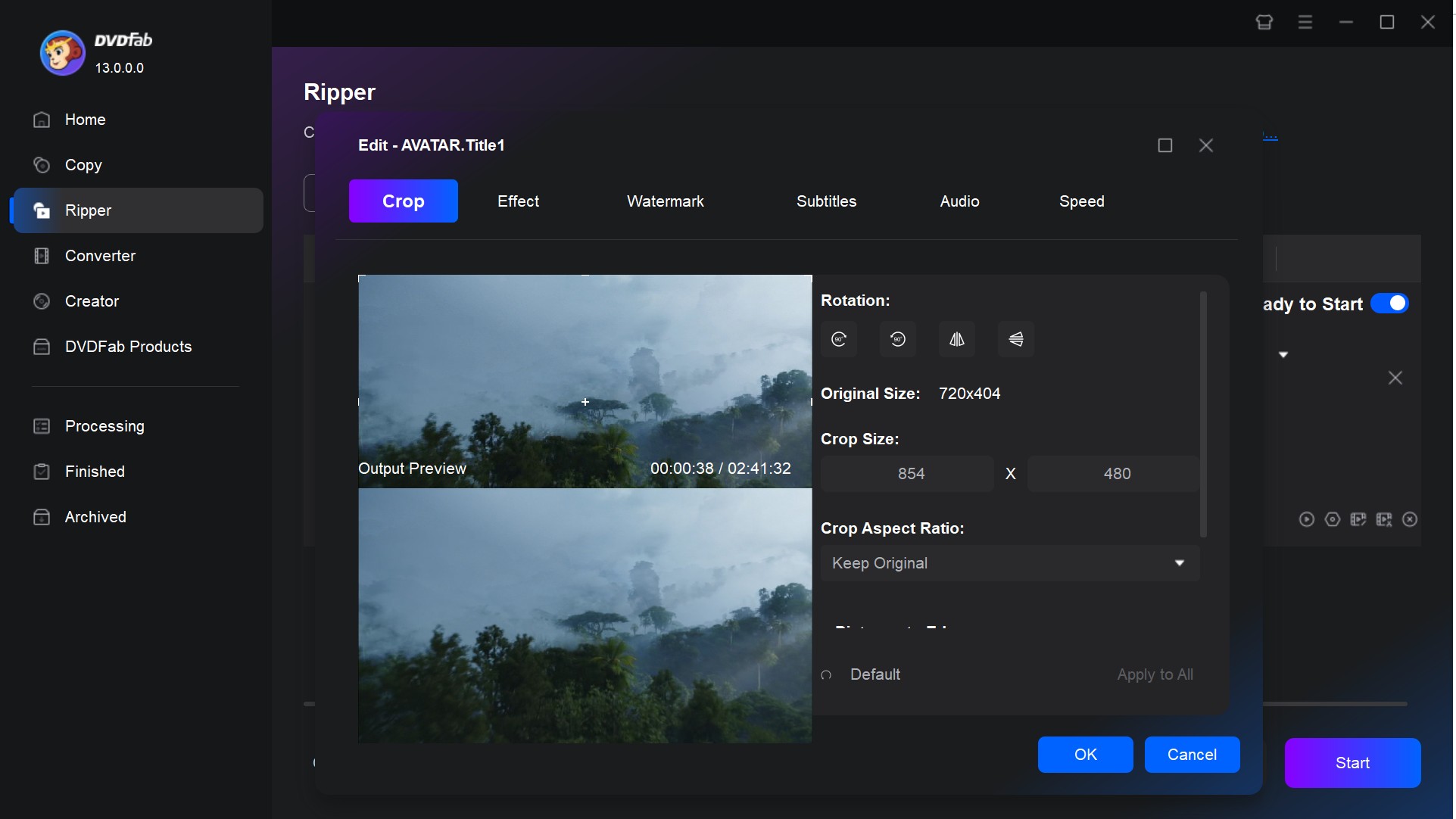Set against a stark black background, this screenshot captures the interface of DVD Fab software. In the upper left corner, "DVD Fab" is displayed in white text next to a blue circle containing a cartoon depiction of a female's head. The left side of the screen features a vertical navigation menu. From top to bottom, the menu items are: Home, Copy, Ripper (highlighted in gray), Converter, Creator, DVD Fab Products, Processing, Finished, and Archived.

On the right side of the screen, the word "Ripper" appears prominently in bold white text. Below "Ripper," various submenu options are listed, including "Edit," "Avatar," and "Title 1." Underneath these, a horizontal menu bar provides further options, each in white text. The options are: Crop (highlighted in a blue box), Effect, Watermark, Subtitles, Audio, and Speed.

In the lower right corner, three blue action buttons are arranged horizontally. The first button reads "OK," followed by a "Cancel" button, and finally a "Start" button. The overall layout is clean and organized, making navigation straightforward for the user.